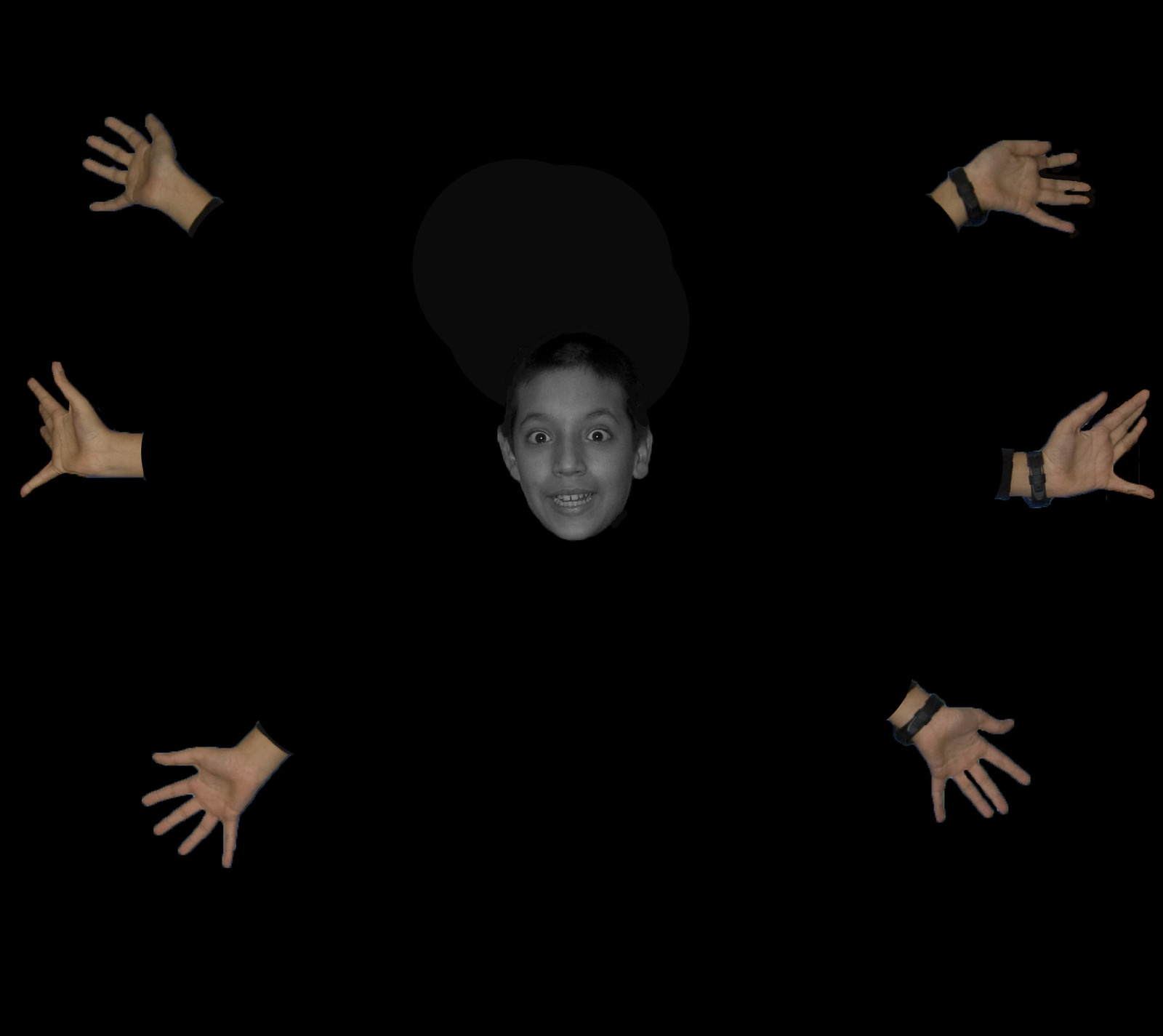In this striking and artistic photograph, set against a deep black background, a young individual with close-cropped brown hair and wide-open brown eyes stares intently at the viewer from the center of the frame. The expression on their face, a blend of surprise with arched eyebrows and a subtle smile, adds to the intrigue. Surrounding their face are six disembodied hands, each extending from the dark void. These hands, likely a composite image or an illusion created by individuals in black clothing, give the illusion that the central figure possesses multiple arms, reminiscent of depictions of Hindu deities. The hands are positioned with one at the top left, one at the middle left, one at the lower left, and their counterparts mirrored on the right side. Each hand is adorned with similar wristbands, reinforcing the sense of symmetry and unity. The dark gray shape hovering above the head adds a subtle accent, making the central figure appear almost ethereal amidst the surreal arrangement. This image fuses elements of photo manipulation and visual illusion, leaving a lasting impression of an almost divine multiplicity.